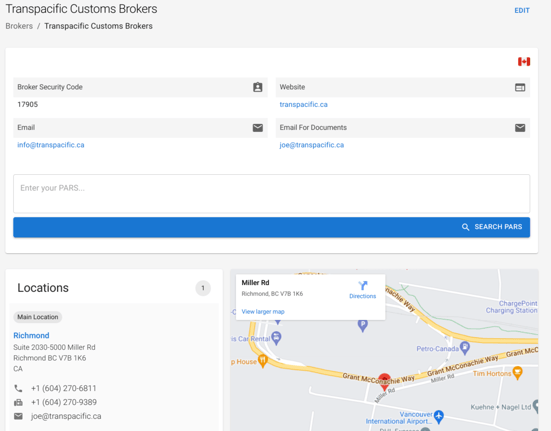The image depicts a webpage layout for Trans-Pacific Customs Brokers. The background is a muted gray, segmented into multiple sections: one larger rectangular section at the top and two smaller sections below.

At the very top, the title "Trans-Pacific Customs Brokers" is prominently displayed in black text. To the right of the title, in smaller blue text, is the word "edit."

Below the heading, the main section features a white box. On the right side of this box, a small red Canadian flag icon is displayed. Adjacent to the flag, the white box is divided into smaller input fields. The first row asks for the "Broker Security Code" on the left and "Website" on the right. Below this, it requests an "Email" on the left and "Email for Documents" on the right.

Further down, beneath the input fields, is detailed information for each:
- Under "Broker Security Code": the number "17905"
- Under "Website": "Trans-Pacifica.ca" in blue, clickable text
- Under "Email": "info@Trans-Pacific.ca"
- Under "Email for Documents": "Joe@Trans-Pacific.ca"

At the very bottom of the main section, there is an input field for entering your PARS (Pre-Arrival Review System) accompanied by a blue search bar labeled "Search PARS" on the right.

The bottom left section lists the main location:
- "Main Location: Richmond"
- The address and phone number are provided, along with the email address.

The bottom right section presents a map highlighting Miller's Road, presumably indicating the location of Trans-Pacific Customs Brokers.

The entire layout is cleanly segmented, providing clear navigation and information for users of the site.